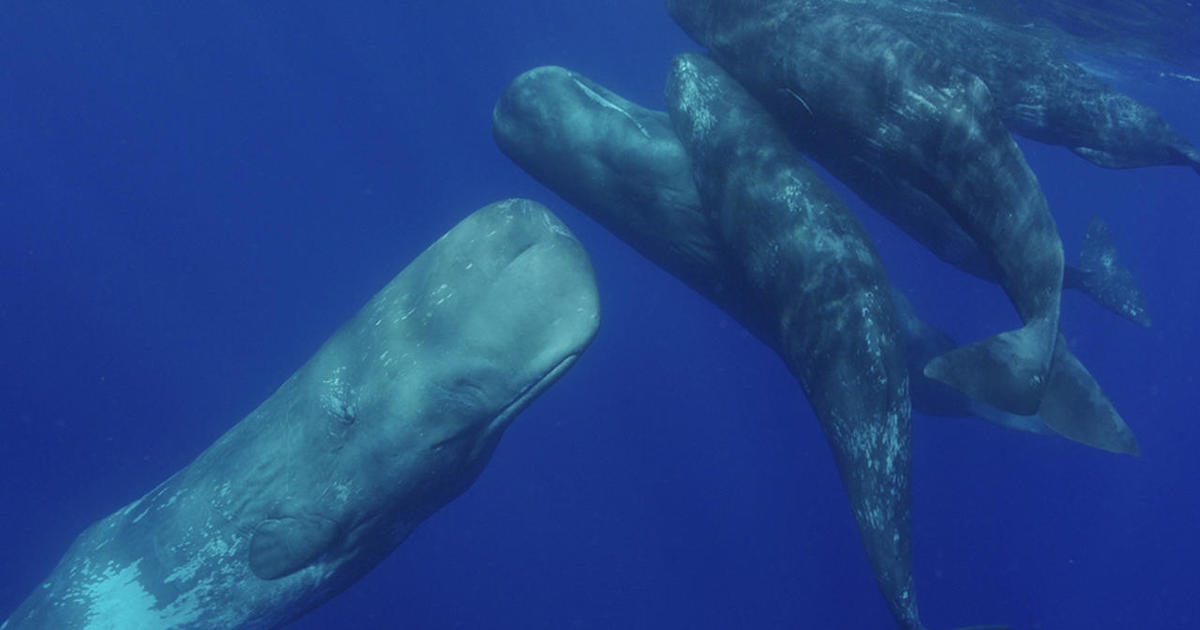In this underwater photograph, we observe a captivating scene set in the deep cobalt blue ocean. The image, which is about twice as wide as it is high, captures a pod of whales, likely sperm whales, gracefully navigating the waters. Dominating the lower left corner, a large whale ascends obliquely, its massive, elongated, cylinder-like body and mottled gray-blue skin highlighted against the deep navy backdrop. Alongside this giant, several smaller whales—presumably calves—swim toward the surface, forming a protective and cohesive group. The whales are distinct with their characteristic elongated snouts and mouths, and their mottled skin glistens faintly. They do not appear to be near the surface, suggesting they are submerged at a significant depth, perhaps over 100 feet, where the sunlight barely penetrates. This serene yet powerful underwater tableau exemplifies the majestic and communal nature of these marine giants.